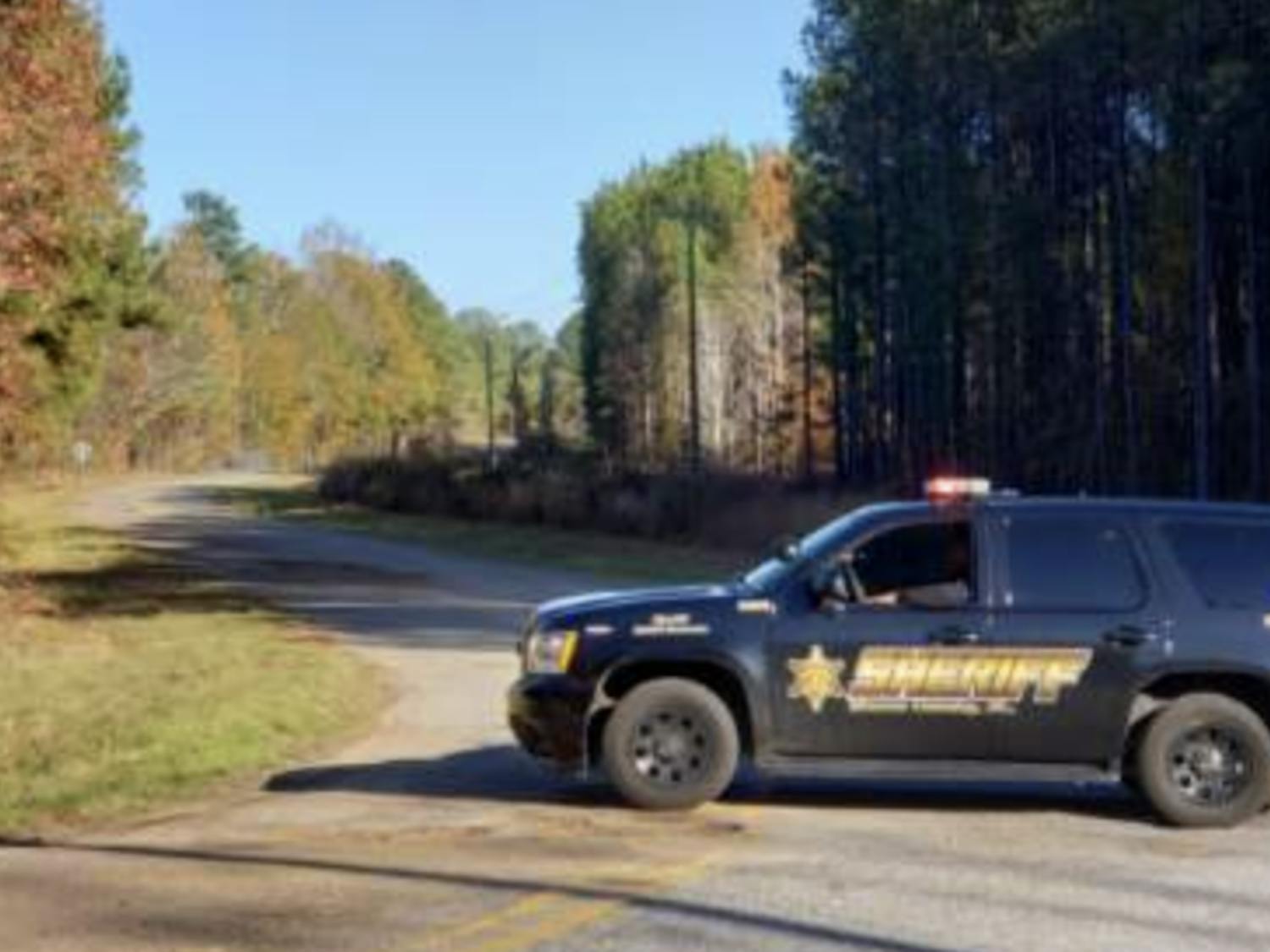A black sheriff's SUV with its red and white lights on is parked horizontally, blocking most of a winding, double-yellow-line cement road. The SUV features a gold star badge and the word "Sheriff" on the driver's side door. The vehicle has black rims and tires, and the driver's window is rolled down with a man in a dark shirt leaning an elbow out. The scene is set on a sunny day with a clear blue sky and the road curving to the left and then back to the right. Tall trees line both sides of the road, exhibiting a mix of green leaves alongside hues of brown, yellow, orange, and reddish tones, reflecting an autumn setting. The photo is a candid, non-professional shot with a slightly grainy quality and not fully in focus.